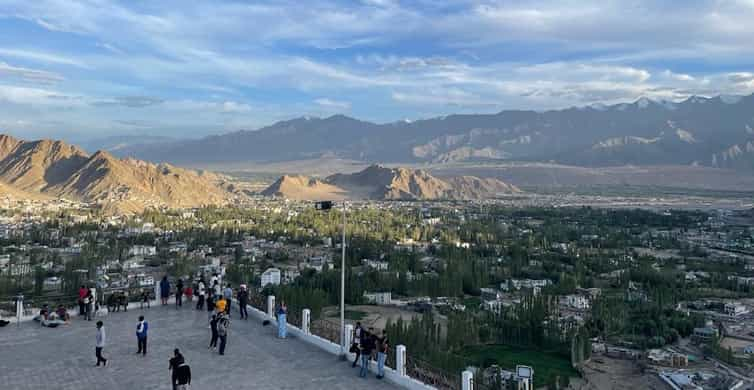This wide-angle overhead shot captures the majestic expanse of the Grand Canyon or a grand mountain range. The foreground features an observation deck in the bottom left corner, enclosed by a white and iron fence, where numerous people are gathered, either gazing at the distant vistas or snapping photographs. Some are positioned near viewfinders to better examine the sweeping panorama. The midground reveals a patchwork of greenery and scattered houses, complemented by tall trees. Further back, the terrain transitions into a desolate, flat desert, leading up to a vast mountain range with some snow-capped peaks on the horizon. The sky is a vivid blue, adorned with wispy white clouds, adding to the serene and expansive feel of the landscape.